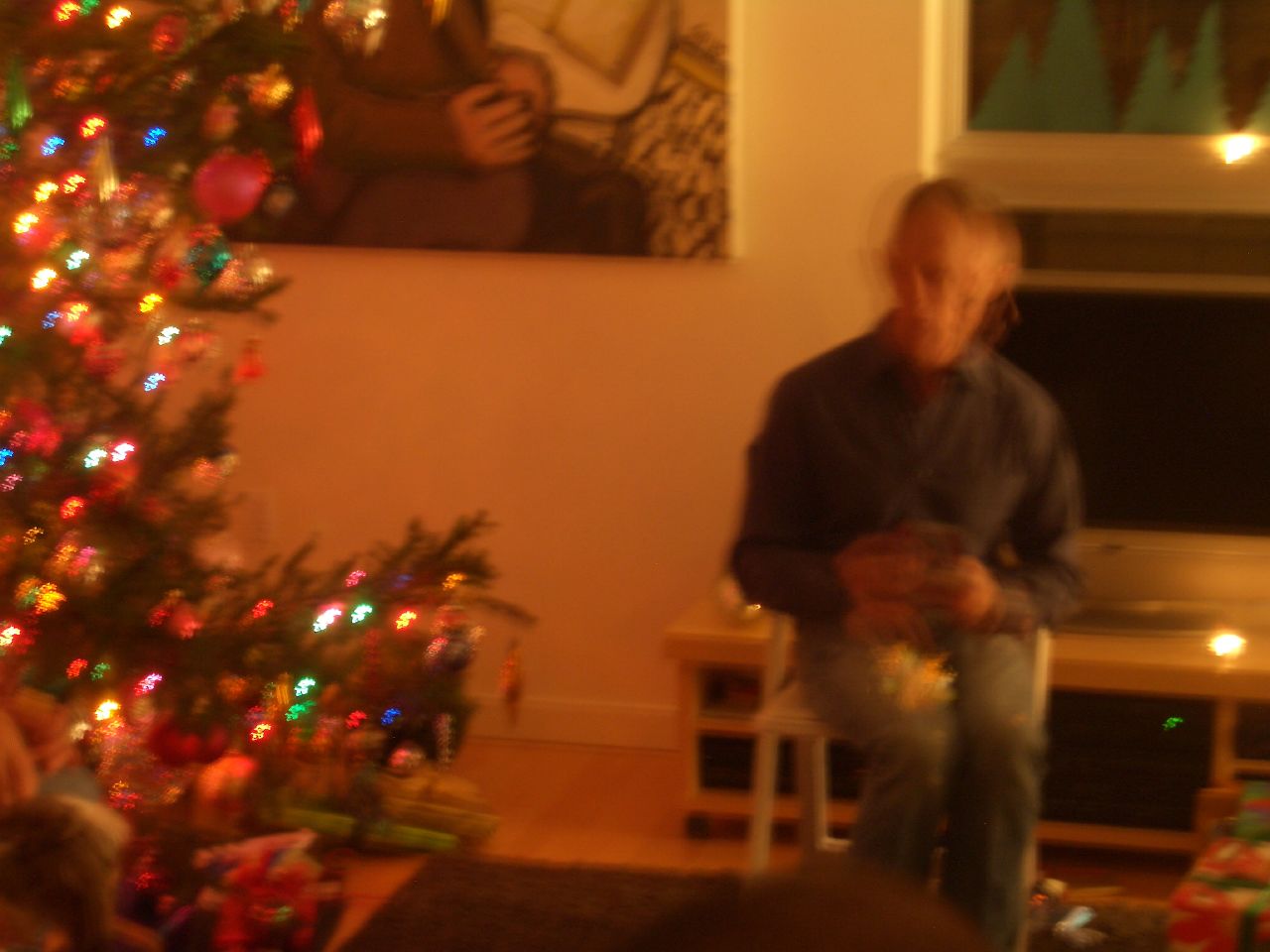A man sits on a white chair in this slightly blurred photo, possibly due to motion from either the subject or the camera. The image, oriented in landscape and only marginally wider than it is tall, captures the man dressed in jeans and a long-sleeved shirt that appears to be either gray or green. He is holding an object that emits various colored lights, likely Christmas lights. His gaze is directed to the left, but a ghostly blur of his face looking to the right indicates movement during the photo capture. The background includes a TV and TV stand, a partially visible painting in the top left corner, and a lit-up Christmas tree adorned with presents beneath it.